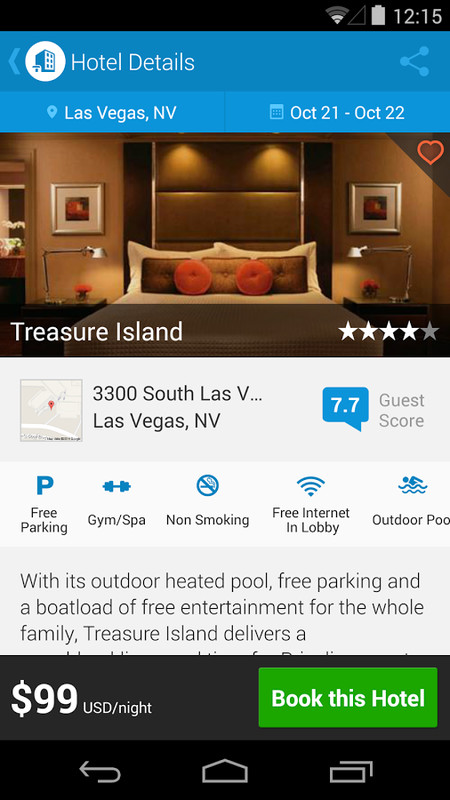Screenshot of Hotel Details for a stay in Las Vegas, Nevada from October 21st to October 22nd, featuring a detailed breakdown of the amenities and booking options. The image shows the device's status bar with the battery level, time, and signal strength. The primary picture is of a well-decorated bedroom. The hotel holds a five-star rating and displays key information such as the address, guest score, available internet, outdoor heated pool, non-smoking policy, gym, spa, and free parking. All these features are available for $99. Additionally, a green button prominently displays "Book Now" next to a description highlighting amenities: "With its outdoor heated pool, free parking, and a host of free entertainment options for the entire family, Treasure Island Delivers." The hotel enjoys four solid stars and is marked with a little heart icon. The interface also includes a home button, a copy button, and a map icon for easy navigation.